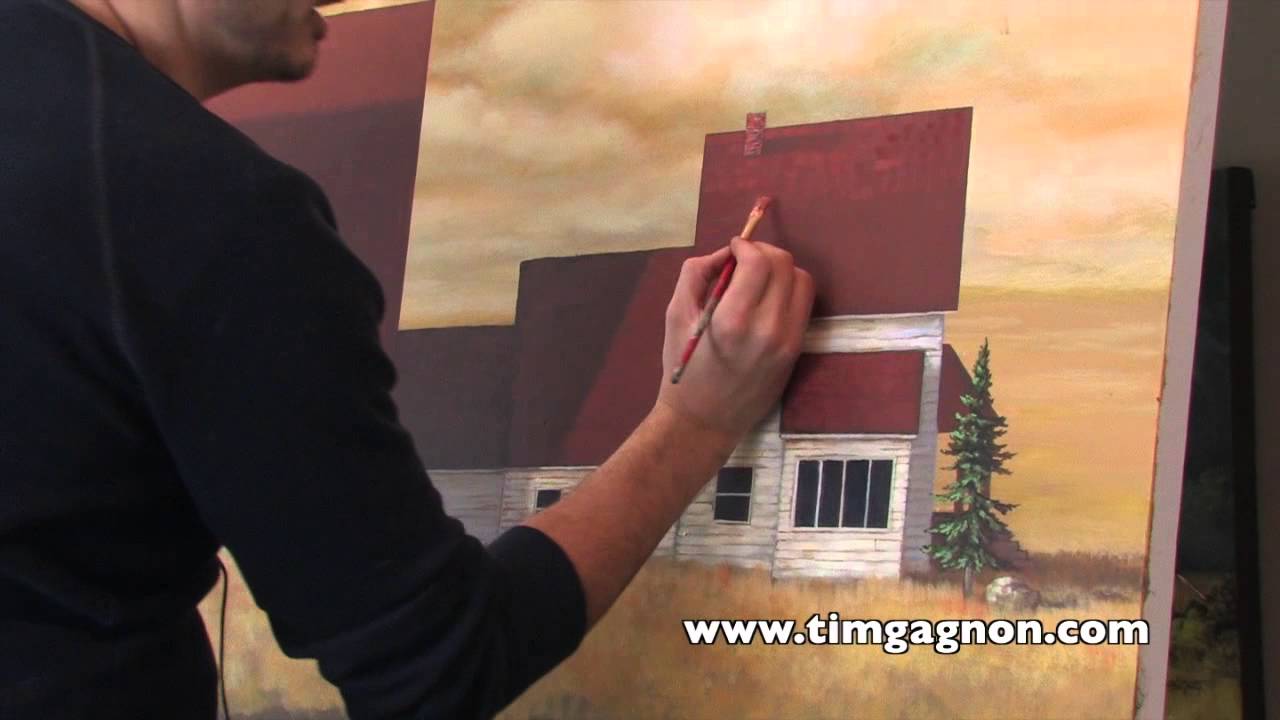The horizontally oriented photograph captures a close-up of an artist engaged in painting a house on a canvas. The artist, a Caucasian male, is positioned on the left side of the image, cropped at the top of his head and the left side of his body. He is wearing a long-sleeved black sweater with the right sleeve rolled up to his elbow, revealing his forearm. His right arm is bent at the elbow, extending outward and upward, with his hand holding a paintbrush against the canvas. The lower half of his face is visible, showing a hint of facial hair.

The focal point of the photograph is the canvas, which features a detailed painting of a farmhouse. The house has a red roof and white horizontal clapboard siding, accented by black rectangular windows. The painting also includes two smaller additions to the left side of the house. On the right side of the house, there is a large evergreen tree, painted with precision. The background of the painting portrays a yellowish, cloudy sky, transitioning into an orangey haze towards the bottom, which represents grassy terrain with hints of greenery. In the bottom right corner of the photograph, white text outlined in black reads "www.timgagnon.com".